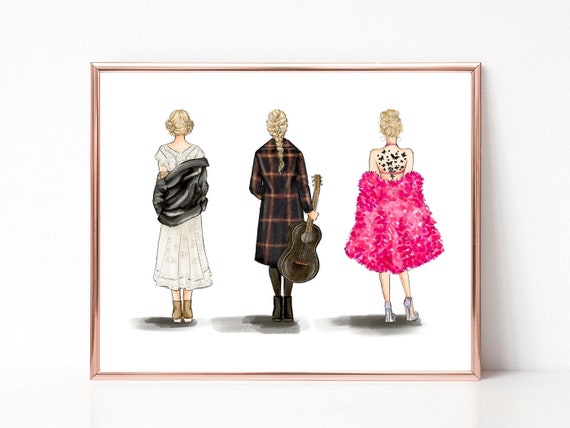The image shows a framed piece of artwork with a glossy, pinkish-gold frame leaning against a white wall on a white surface. Inside the frame, the artwork depicts three women standing with their backs to us. Their shadows are cast on the ground beneath them, adding depth to the scene. 

On the left, the first woman is wearing a white dress that falls just above her shins, paired with brown socks and white sandals. She has short blonde hair and is in the process of removing a black coat from her shoulders.

In the center, the second woman, who has long blonde hair braided down her back, is wearing a black coat with a checkered pattern outlined by red stripes. She is holding a brown guitar behind her back.

To the right, the third woman is adorned in a black and white spotted crop top and white high heels. With a pink shawl draped over her shoulders, she appears to be taking it off. Her blonde hair is styled in a bun, and she has tattoos of black butterfly designs on her back.

Together, these elements create a striking and detailed representation of fashion and poise captured in the artwork.